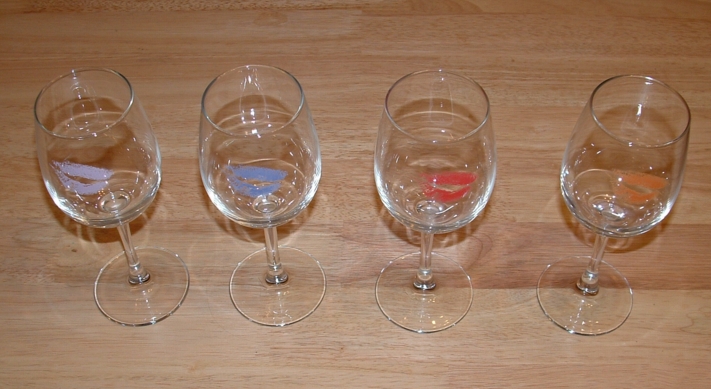This photograph captures a close-up view of four clear wine glasses aligned in a row on a light brown wooden table with horizontal wood grain. Each glass, identical in design with a clear base and stem, contains a liquid that appears to be water, based on its colorlessness and clarity. The image is taken from a slightly elevated angle, revealing both the tops and sides of the glasses. Prominently, each glass bears a distinct colored lipstick imprint positioned on the middle of the side, as though kissed. The imprints progress from left to right with the first glass showing purple lips, the second blue, the third red, and the fourth orange. Light reflections are visible on all glasses, hinting at the light source from the room or camera flash. There is a small space between each glass, enhancing the clarity of each colored lip print.